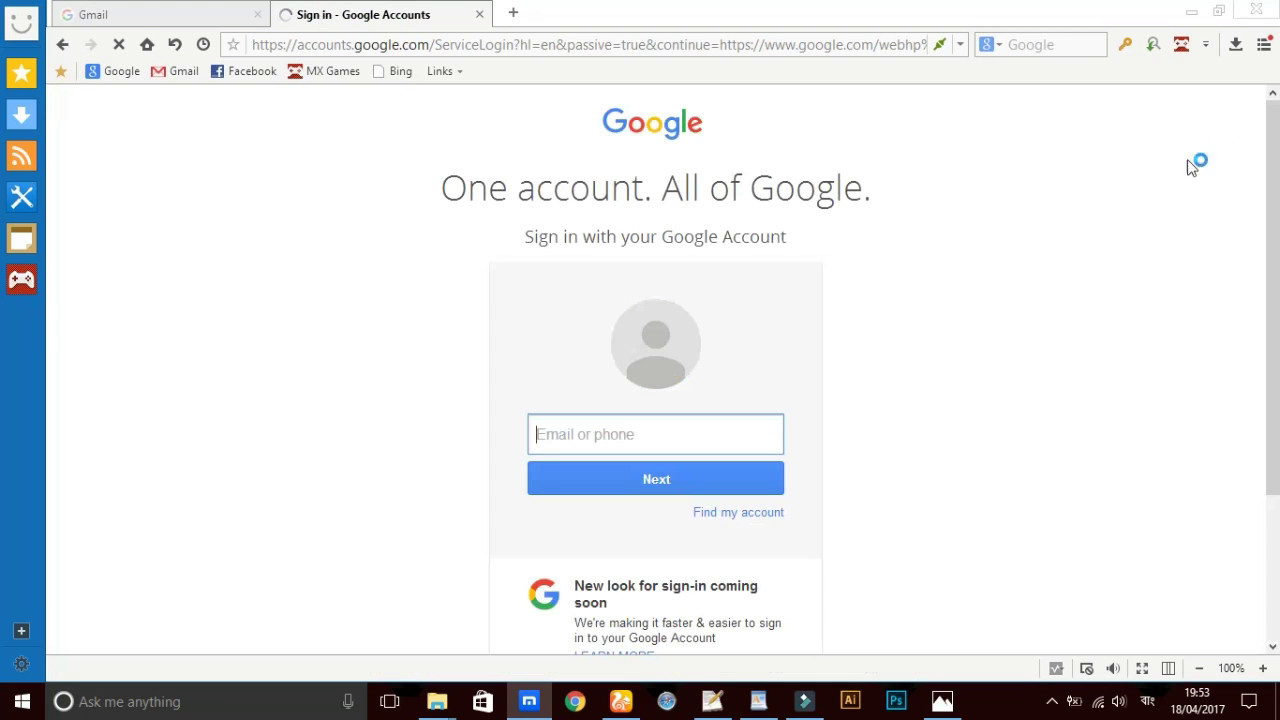In this image, we see a web browser with two open tabs. The first tab displays Gmail, and the second tab is open to the Google Account sign-in page at accounts.google.com. On the left side of the browser, there is a blue vertical strip containing several icons: a start icon, a shopping icon, a download icon, a connection icon, a gear or settings icon, and a game console icon. 

At the center of the image, the Google sign-in page is prominently displayed. It features the Google logo, the text "One account. All of Google," and instructions to "Sign in with your Google Account." Below this text, there is a field for entering an email or phone number, a "Next" button, a "Find my account" option, and a note indicating that a new look for the sign-in page is coming soon, promising a faster and easier sign-in experience.

At the bottom of the image, the Windows 10 taskbar is visible. On the far left, we can see the Windows icon, while on the far right, there are status bar icons. In the center of the taskbar, several application icons are displayed.